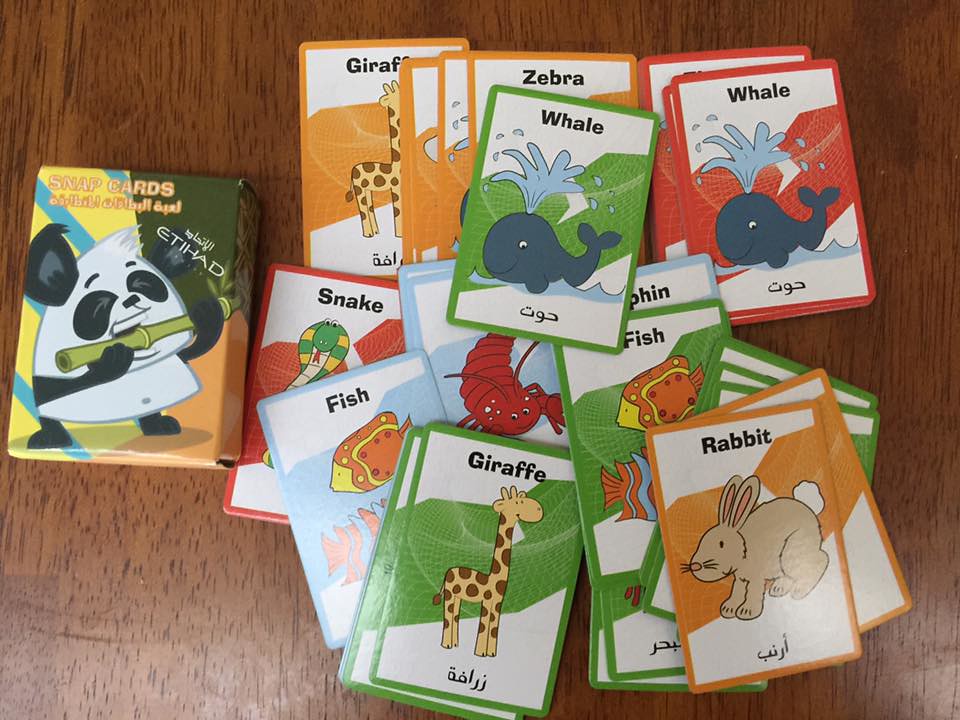In an indoor setting, we see a colorful array of "Snap Cards" laid out across a wooden table, designed as a children's game to teach animal names and possibly multiple languages. The game features a mix of animals like giraffes, whales, zebras, dolphins, fish, lobsters, snakes, and rabbits, each illustrated comically with their own distinct color—green, red, orange, and blue. The cover of the game box showcases a panda playing a bamboo flute, hinting at the playful nature of the game. Some text on the cards appears to be in a non-English language, possibly Middle Eastern, adding an educational layer. The cards are scattered about, suggesting an engaging and interactive game that's perfect for young children.